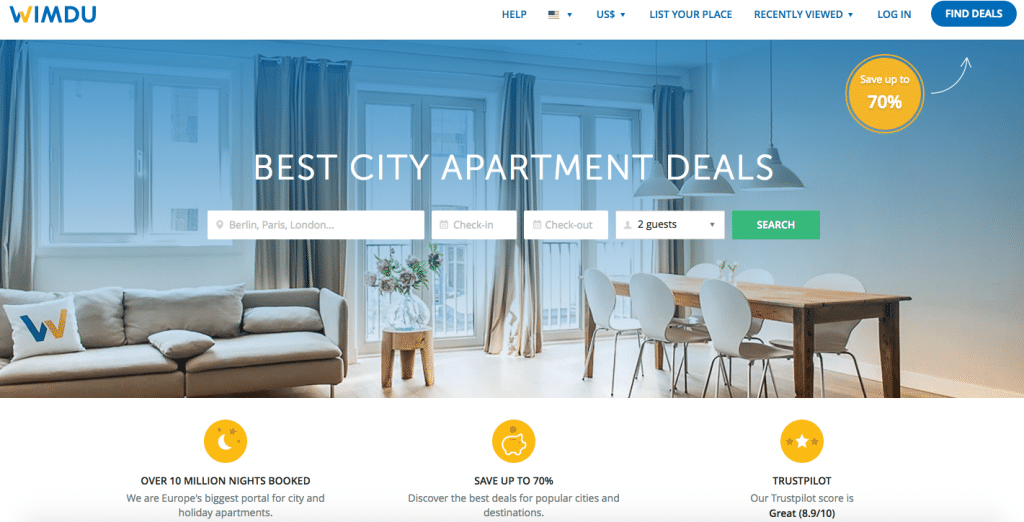The image depicts a platform named Wimdu, with a distinct logo where half of the "W" is colored in blue, the other half in yellow, and the rest of the text is in blue. Below the logo, there are navigation options including 'Help,' an icon of the U.S. flag, a dropdown for selecting the U.S. dollar currency, and links for 'List Your Place,' 'Recently Viewed,' 'Log In,' and 'Find Deals.' Prominently displayed is a circle highlighting the message "Save up to 70%." A notable mention states, "For 10 million nights booked, we are Europe's biggest portal for city and holiday apartments." The image further promotes saving up to 70% on accommodations, urging users to discover the best deals in popular cities and destinations, boasting an impressive TrustPilot score of 8.9 out of 10. The accompanying picture is of an apartment featuring large, floor-to-ceiling windows, a long dining table set for six, a contemporary couch, and a coffee table adorned with a large vase filled with greenery.